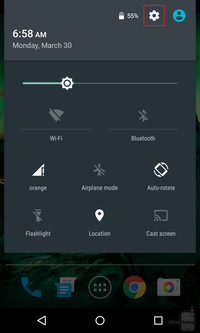A detailed screenshot of a smartphone interface, slightly cropped on all sides, revealing various on-screen elements. At the top left, the time is prominently displayed in bold white text as "6:58 AM", below which the date "Monday, March 30th" appears in grey. On the top right, a battery icon indicating 55% charge is displayed next to a white gear symbol enclosed in a red rectangle. Adjacent to this, a cyan blue silhouette of a person with a black circular outline denotes a profile picture.

Below the status bar, a quick settings panel features several toggles, most of which are greyed out. A sun-like icon with blue teardrop adjustments likely represents brightness controls. The Wi-Fi and Bluetooth symbols both have lines through them, indicating they are off. The cell signal strength icon, marked with an exclamation point and labeled "Orange", appears in white.

Further icons in this panel include a greyed-out airplane mode, auto-rotate symbolized by two half circles, and an off flashlight icon with a line through it. A location pin (GPS), however, is white, signifying it is active. Additionally, a cast screen icon featuring a square with a sideways Wi-Fi signal is visible.

On the bottom of the screen, a dock contains various app shortcuts: a blue phone icon for dialing, two overlapping pieces of paper (one dark blue and one grey) represent chatting, with respective white and black lines. At the center, a circle with six dots signifies accessing additional apps not present on the home screen.

The Google Chrome icon is also on display, featuring distinct segments in green, red, and yellow converging on a thin white circle with a dark blue center. Lastly, a colorful folder, encircled by shades of yellow, orange, red, blue, purple, and green, is present. The bottom bezel houses white navigation buttons: a left-facing triangle, a circle, and a square.